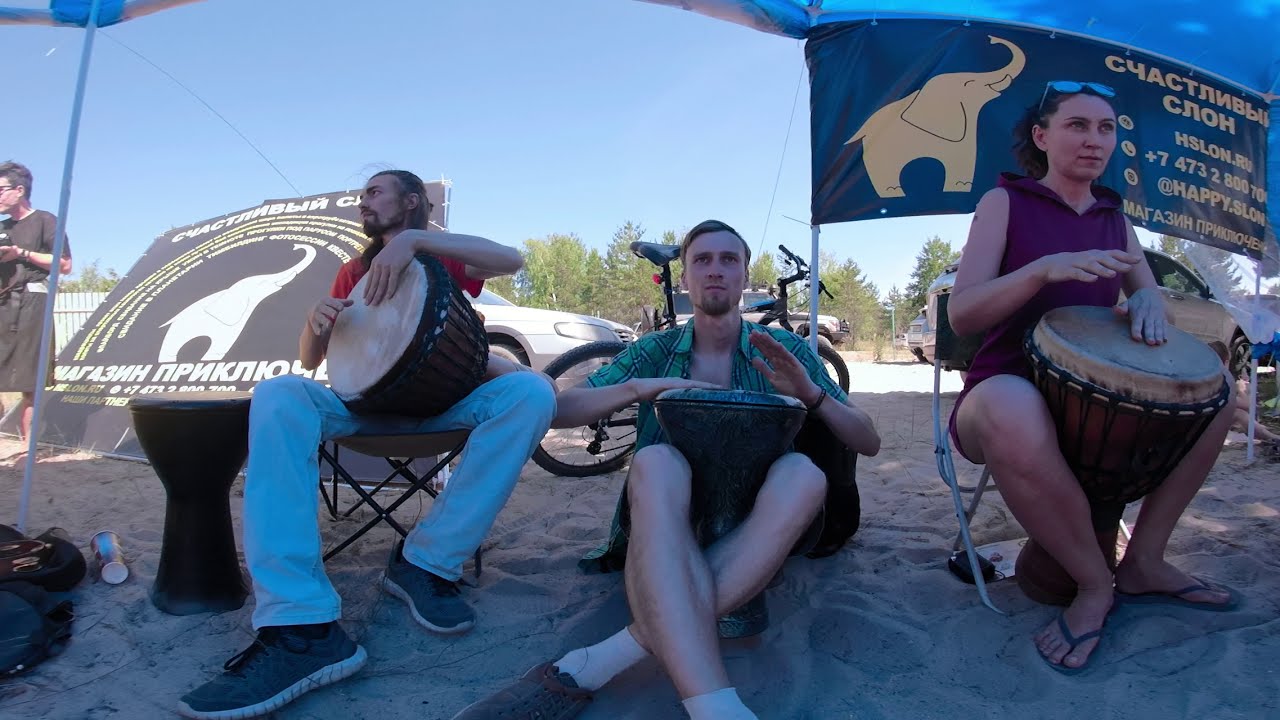On a bright, sunny day at the beach, three musicians sit in a row, deeply engaged in playing bongo drums. Behind them, black and blue banners with images of elephants and text in a foreign language, likely Russian, flutter in the breeze. The text on the banners, in gold and white lettering, includes contact details and possibly an email address. A bicycle is also visible in the background, along with parked cars and lush green trees against the clear blue sky.

In the center, a white man with a goatee and short brown hair sits cross-legged on the sandy ground, playing a black bongo drum. He wears a green, unbuttoned, checkered shirt, shorts, white socks, and black sneakers.

To his right, a woman with short brown hair, tied back, is perched on a folding chair. She sports a purple sleeveless top, shorts, flip-flops, and sunglasses resting on her head. She plays a maroon percussion instrument, her neutral expression focused on the music.

On the left, another man, slightly dark-skinned with a neatly trimmed beard and long hair, sits on a chair, playing a drum on his lap. He wears a red t-shirt, light blue jeans, and gray sneakers, and gazes contemplatively to his right. In the far left of the image, there is an unattended bongo drum with a pair of sunglasses on the sand beside it, and a person standing, wearing a black gown-like outfit. The scene is lively yet serene, encapsulated by the rhythmic drumming and the natural, tranquil backdrop.